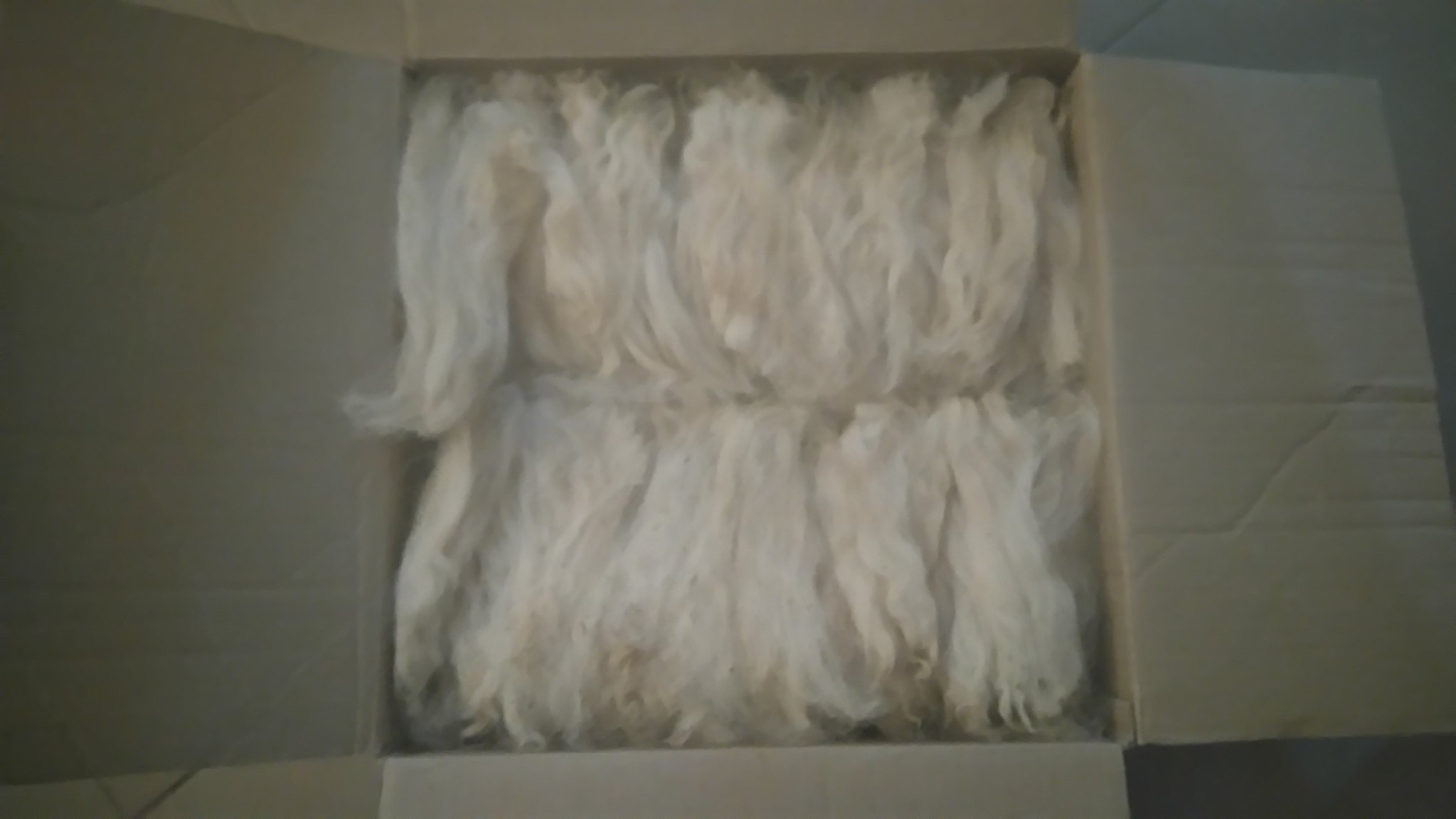A blurred, dimly-lit photograph depicts a large brown cardboard box, square in shape, with its flaps bent outward. Inside the box, which is viewed from a top-down angle, are two orderly rows of white wool or a similar natural textile, such as sheep or angora goat wool. The wool looks manicured and soft, with a slightly rippled texture and curly tips, appearing clean and pristinely lined up. The wool is relatively straight, giving an impression of being quite neat. The box flaps obscure some of the surroundings, but there are hints of a plain white tile floor with darker grout visible in the top corners of the image. The cardboard box itself shows some folds and corrugations, especially at the edges.